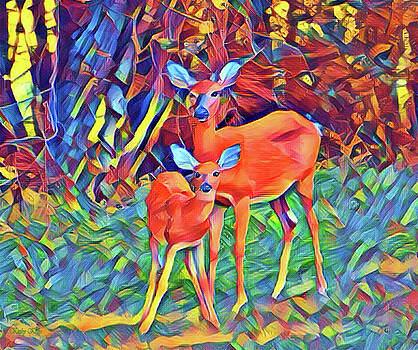The image appears to be an artistic depiction, potentially a painting, of two deer standing amidst a vibrant, colorful background. The adult deer, positioned on the right, is accompanied by a juvenile deer slightly to its left. Both deer are staring directly at the viewer with their ears perked up, emanating a sense of alertness. Their bodies exhibit a combination of gray and brown hues, with their legs transitioning from brown to yellowish tones toward their bottoms. The deer have striking black eyes and noses. 

The background is a vivid mosaic of colors and patterns, with a distinct division; the upper portion of the image showcases deep, intense colors like yellow, blue, red, and gray zigzag lines, while the lower portion fades into lighter shades of blue, green, and light brown. The entire scene is reminiscent of a forest setting but rendered in a psychedelic, almost surreal manner, with rainbow-like foliage and fantastical multicolored accents. This highly detailed, non-realistic portrayal of nature creates a striking contrast between the natural subjects and their fantastical environment.